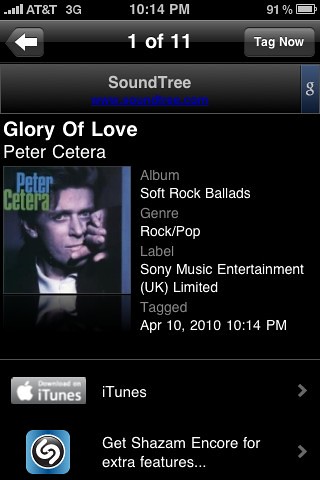The image is a screenshot of someone's iPhone displaying their iTunes interface. The time at the top of the phone is 10:14 p.m., the battery is charged to 91%, and the network provider is AT&T. The screen shows that the user is listening to "Glory of Love" by Peter Cetera, which is the first song in a playlist of 11 tracks. The album cover is visible on the left side of the screen and features the name "Peter Cetera" in blue and green font, with Peter leaning against a doorframe looking concerned. The album is titled "Soft Rock Ballads," categorized in the Pop Rock genre, and released under Sony Music Entertainment UK Limited. This track was tagged on April 10, 2010, at 10:14 p.m. All the text information, such as the album, genre, label, and tagging date, is displayed in white lettering, while the titles are in gray. Additionally, there are links to iTunes and Shazam with their respective logos at the bottom of the screen.